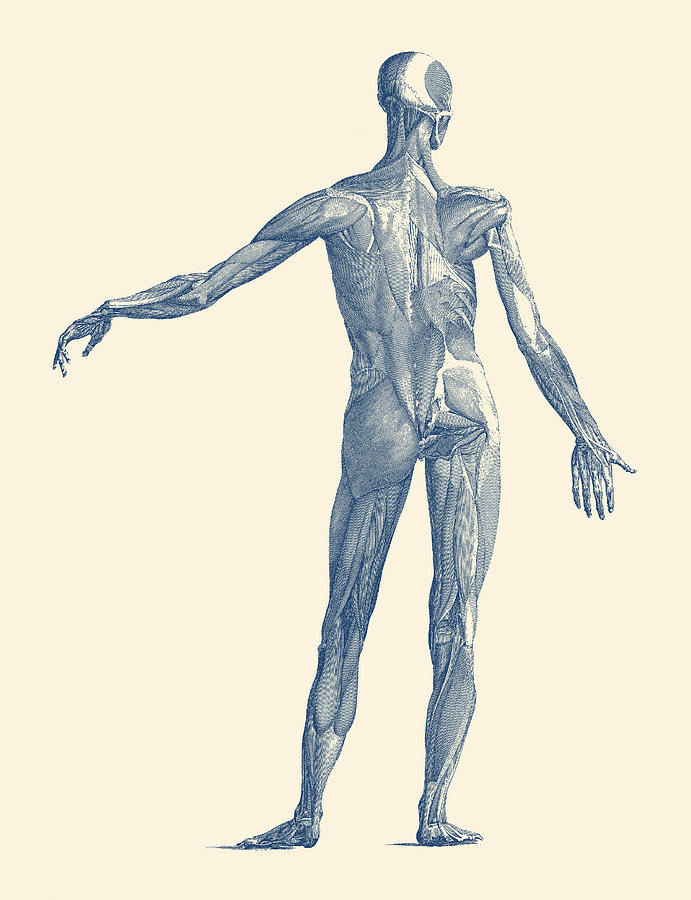The image is an intricate, blue scale illustration of the human body with the skin removed to reveal various muscle groups. The figure is depicted from the back, showcasing an array of muscles including the quadriceps, gluteal muscles, trapezius, deltoids, hamstrings, and the intricate back muscles. The shoulder blades and plantar muscles of the feet are prominently visible. The background is light gray, with the illustration seeming to be printed in blue ink.

The figure stands flat on both feet, slightly leaning to the right so that the right hip juts out. The head is turned slightly to the right, allowing a partial view of the back right of the head. The left arm extends nearly parallel to the ground, with some fingers curled and the thumb facing forward. In contrast, the right arm bends oddly at the upper arm, held at a 45-degree angle to the side as if the thumb is hitchhiking. The left leg displays a side view, while the right leg shows the back of the leg, enhancing the detailed representation of the muscle anatomy.

Overall, the human body in this image is a testament to the complexity and artistry of the muscular system, primarily displayed in beige and bluish-black hues.